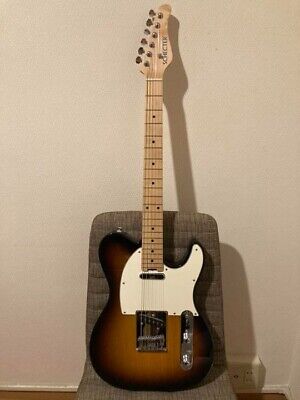This color photograph features an electric guitar prominently displayed on a light brown chair, which lacks armrests, positioned against a slightly off-white, cream-colored wall. The guitar, boasting a rock star look, has a body with a light brown and dark brown outline, complemented by a white pickguard. The guitar’s neck is made of a light-colored wood and is adorned with black strings and dot inlays that guide the length of the neck. Notably, two dots are positioned near the center of the neck, just above the chair. At the headstock of the guitar, there are six silver tuning knobs, each connected to the strings. There's also some writing on the right side of the headstock that hints at the brand, possibly beginning with an "S," but it's too small to discern clearly. The background reveals a wooden-finished floor, a wall outlet, and a fabric element on the chair, possibly dark gray. The guitar casts a light gray shadow against the wall, adding depth to the image.